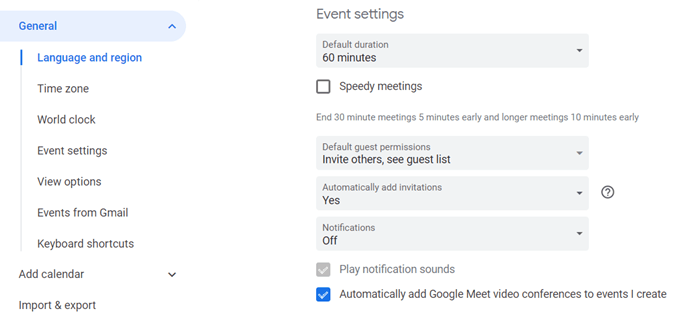Here's the refined and detailed caption:

"A screenshot from a Windows interface displayed on a white background. On the left side of the screen, there is a light blue tab labeled 'General' in dark blue text at the top, accompanied by an upward-pointing arrow to its right. Below this tab, a list of settings is presented in dark blue text, starting with 'Language and Region.' The remaining settings are listed in black text as follows: 'Time Zone,' 'World Clock,' 'Event Settings,' 'View Options,' 'Events from Gmail,' 'Keyboard Shortcuts,' 'Add Calendar,' and 'Import and Export.'

On the right side of the screen, within the 'Event Settings' section, there is a drop-down menu displaying 'Default duration 60 minutes.' Below this menu, a check box labeled 'Speedy Meetings' is present with a brief explanation beside it: 'End 30-minute meetings 5 minutes early, and longer meetings 10 minutes early.' Further down, another light gray drop-down box indicates 'Default guest permissions,' with options such as 'Invite others' and 'See guest list.' Finally, an additional light gray drop-down box shows 'Automatically add invitations,' which repeatedly lists 'Yes.'

Overall, the image represents an organized settings interface in a Windows environment, detailing various configurable options related to event scheduling, permissions, and calendar management."